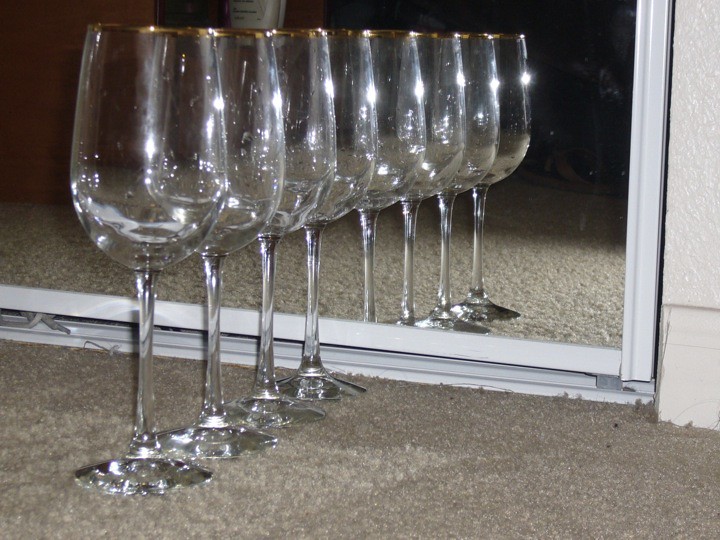The photograph showcases a meticulously arranged row of four identical clear wine glasses, each adorned with a delicate gold rim at the lip. These glasses, characterized by their long, slender stems and circular bases, are precisely aligned one behind the other, giving an impression of continuity. They are positioned in front of a large mirrored closet door with a white frame, set against a cream-colored, low-pile carpet, suggesting a domestic setting.

The reflection in the mirror creates an optical illusion, making it appear as if there are eight glasses instead of just four. This visual doubling effect is highlighted by the clarity of the mirror, which perfectly replicates the four glasses in an uninterrupted line. The photograph is taken with a flash, causing some glare and capturing subtle details in the background such as a brown sandal and the faint outline of a wooden cabinet, though these elements remain indistinct due to the shadows beyond the flash's reach. Additionally, part of a shoelace peeks out from beneath the closet door, adding a touch of everyday realism to the otherwise elegant composition.